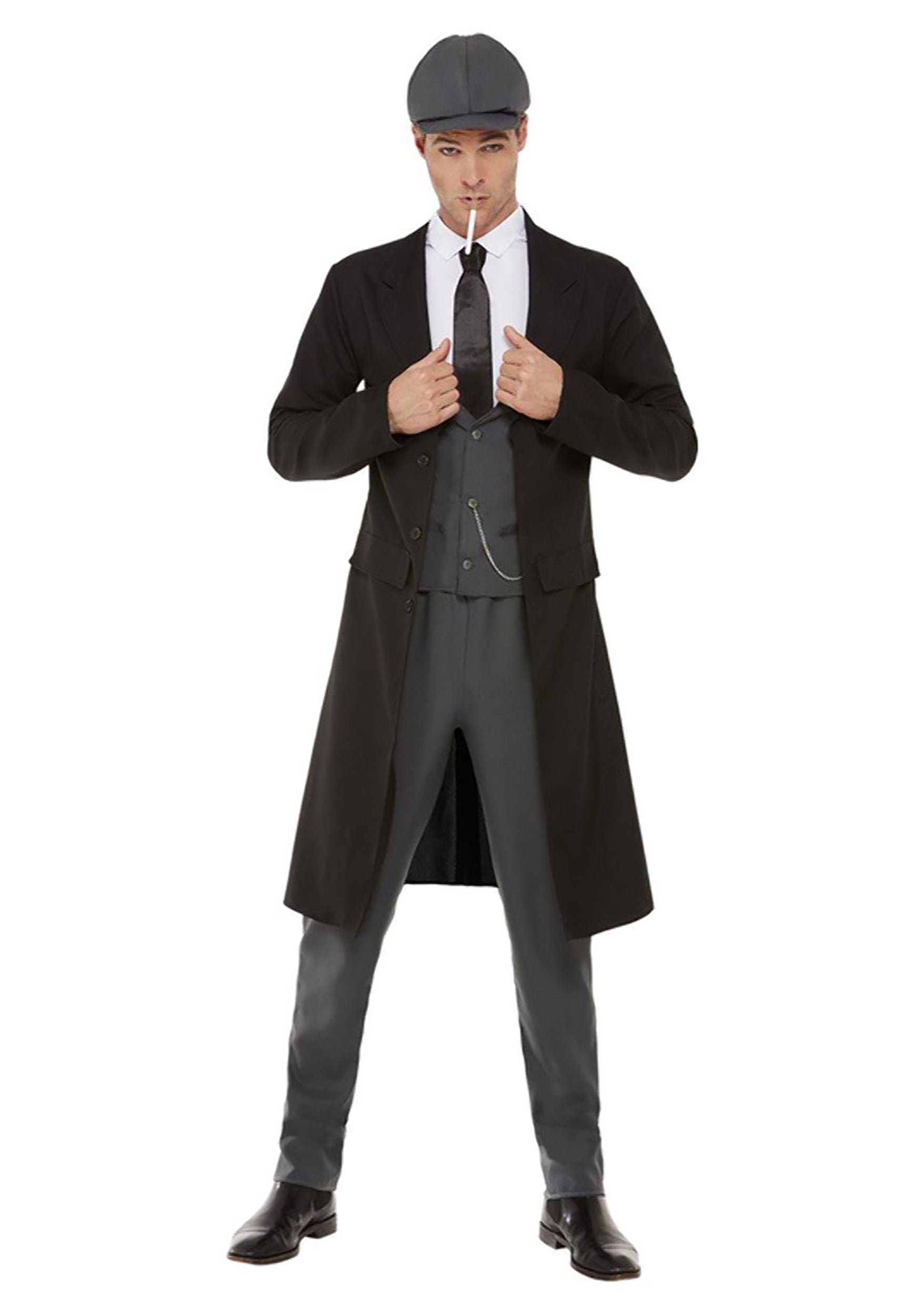The image depicts a man dressed in a formal, somewhat old-fashioned attire reminiscent of a stock photo or a costume from a Halloween shop. He is wearing a long black coat that resembles a suit jacket material, layered over a dark gray waistcoat and a white button-up shirt paired with a black tie that has a noticeable sheen. His ensemble is completed with matching dark gray slacks and black shoes, specifically black Chelsea boots. The man has a paperboy delivery hat or gray boulders cap on his head, obscuring his hair, and he is sporting a cigarette in his mouth. Notably, he has an unusual facial feature of three eyebrows—two on the left side and one on the right—suggesting the image might be AI-generated. He has blue eyes and brown eyebrows, and his seductive gaze is directed at the camera while his head is tilted down. A silver chain is visible on his waistcoat, connecting from a button to a pocket. He is striking a pose with both hands holding the inside of his coat’s lapels, projecting a mood that is both stylish and enigmatic.